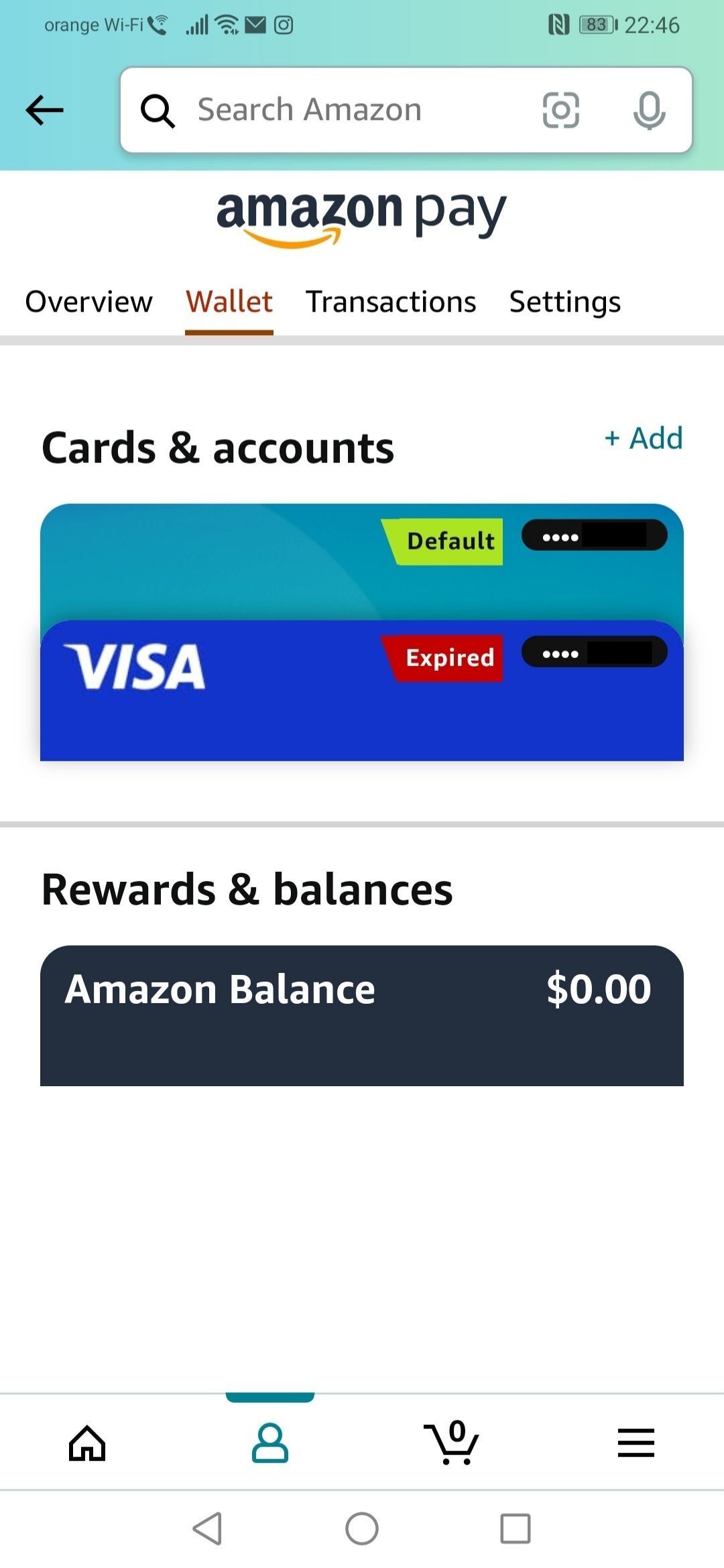The image depicts a smartphone screen showing the Amazon Pay section of someone's Amazon account. At the top, the status bar displays "Orange Wi-Fi," a phone icon, signal bars, a Wi-Fi icon, a mail icon, and the battery percentage indicating 83% at 22:46 hours.

The main interface features an Amazon search bar at the top, followed by icons and tabs labeled Amazon Pay, Overview, Wallet, Transactions, Settings, and Cards & Accounts. The 'Wallet' section is highlighted with a brown underline, indicating it is the current view. 

In the wallet, there is a detailed display of linked payment methods. The default card is a light green card. Another card is a blue Visa card, marked with a red label indicating it is expired.

Further down, there’s a section titled "Rewards and Balances" which shows an Amazon balance of $0.00. At the bottom of the screen, there are navigation icons: "Home," "You," "Cart," and a menu button represented by three stacked horizontal bars. Below these, there are standard Android navigation buttons: a left arrow (back), a circle (home), and a square (recent apps).

The color scheme includes shades of blue, red, green, teal, black, brown, yellow, and white, visually distinguishing different sections and elements on the screen.